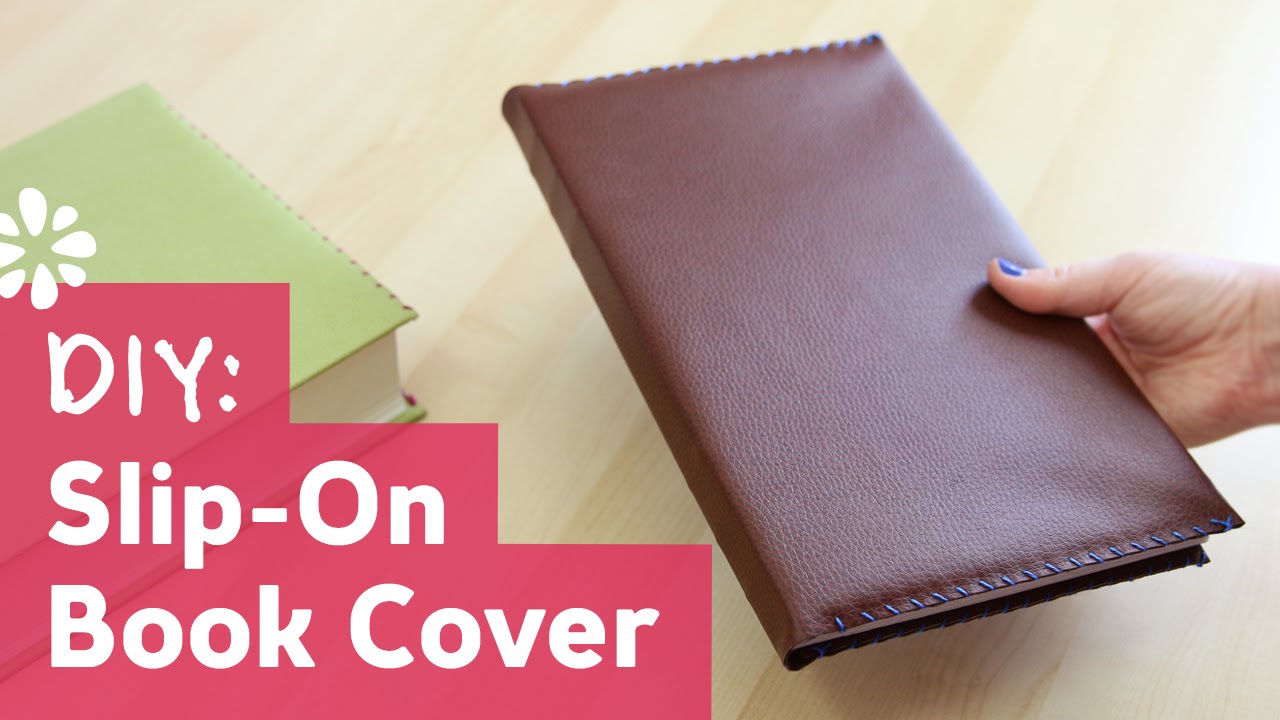In this image, the centerpiece is a woman's hand, distinguished by her blue nail polish, holding a book with a brown leather-like slip-on cover. The cover, designed for protection and aesthetic purposes, features blue stitching along its top and bottom edges. Her thumb is prominently visible while the rest of her fingers are behind the book. To the left, another book with a similar slip-on cover in green can be seen. This entire scene is set against a light wooden tabletop background. Overlaying the image in the bottom left corner, a series of semi-transparent pink boxes house the white text "DIY slip-on book cover," with "DIY" written in a more playful, messy font. Just above this text is a white graphic resembling a flower or an explosion, adding an extra decorative element to the composition.